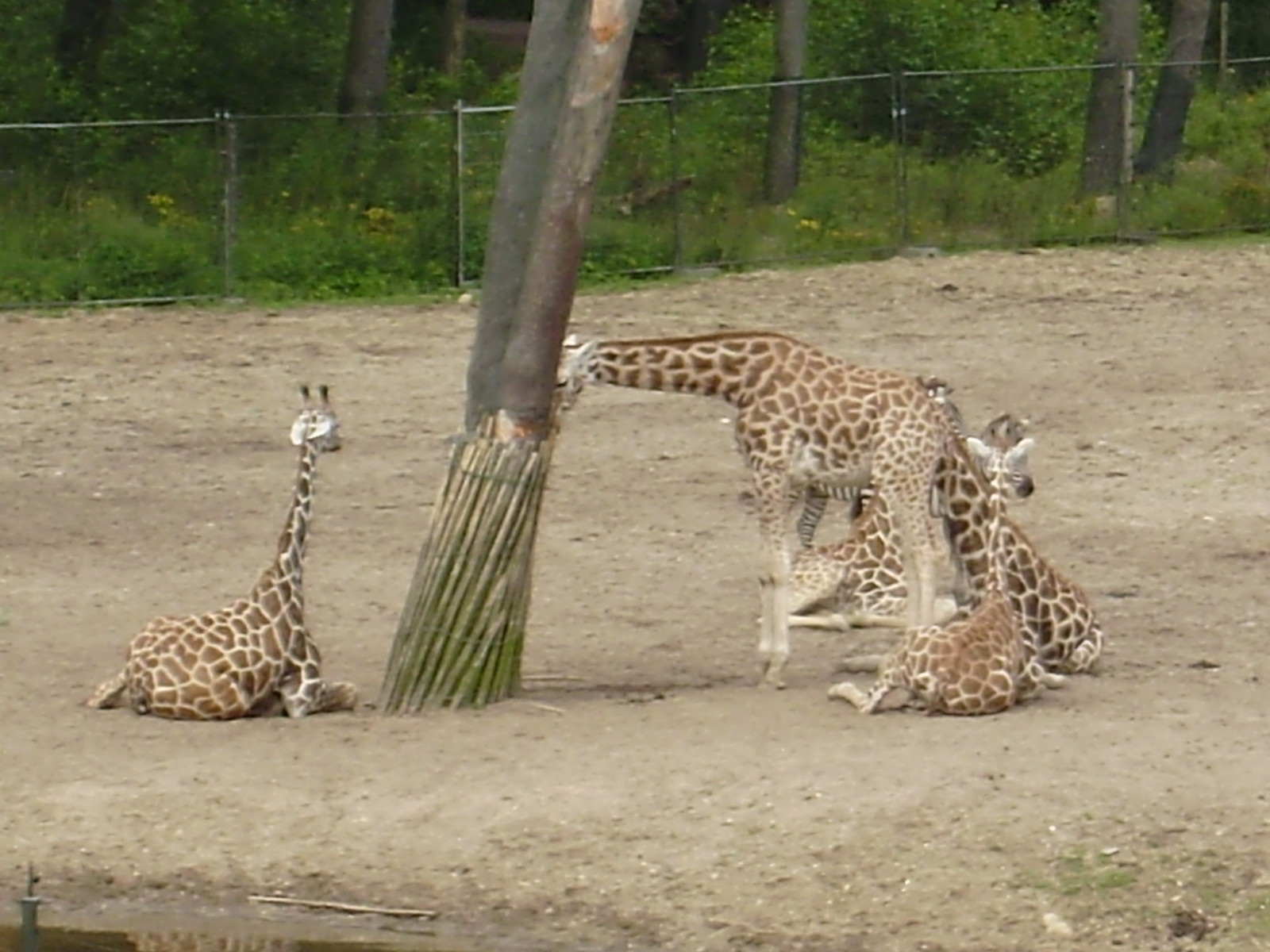The photograph captures a family of giraffes within a zoo enclosure. The scene features a large mother giraffe standing and feeding from the bamboo-wrapped trunks of two trees situated slightly to the left in the foreground. Surrounding her are four to five younger giraffes lounging in the sandy, rocky dirt. These young giraffes have their backs turned to the camera, and one is positioned to the right, while another appears to be looking straight at the camera. The giraffes exhibit their characteristic tan coats with reddish patches and cream-colored bellies, along with distinctive long necks and slender legs. The enclosure is bordered by a chain-link fence, beyond which lies a dense backdrop of trees, brush, and some yellow wildflowers, indicating a wooded area behind the zoo habitat. The trees in the enclosure show signs of being eaten, with missing bark and protective wire around the bamboo stalks at their bases.